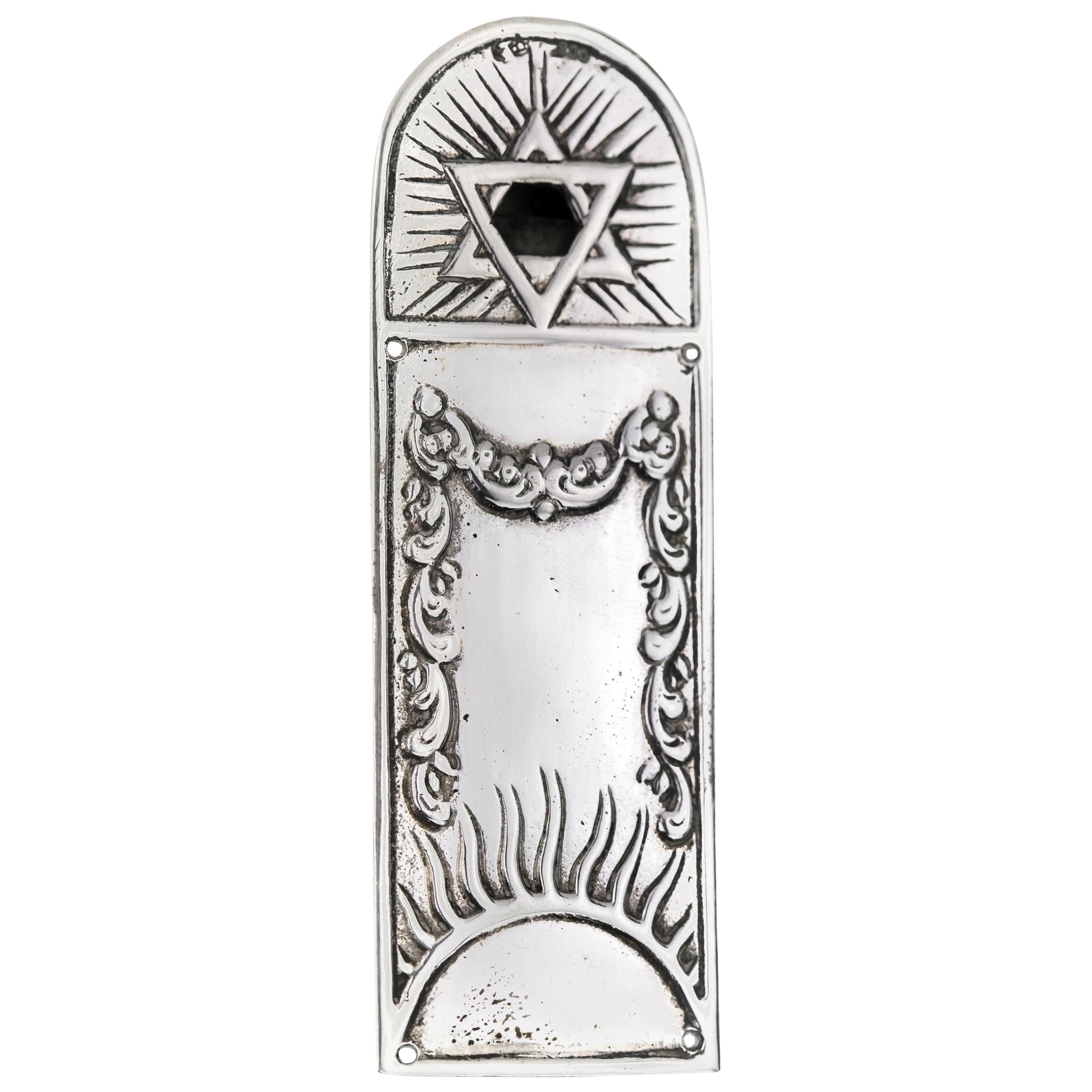This image portrays an antique silver metal artifact, likely of Jewish religious significance, featuring an intricate design suggestive of a doorway or ornamental wall piece. The object, tarnished yet in good condition, vertically elongates into a curved arch at its top. The upper section showcases a prominent Star of David, emitting radiant lines, which signifies illumination or reverence. Below this, a stylized hanging vine or garland extends across the piece, lending an elegant frame to the design. The bottom half of the artifact features a radiant sun motif, adding to the symbolic richness of the piece. Notably, the artifact includes holes, perhaps intended for hanging it on a wall. The entire object, composed of tarnished but well-preserved silver, radiates historical and religious importance.